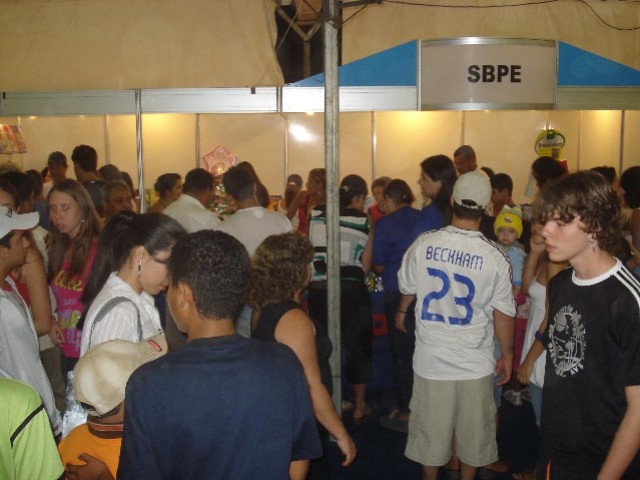This rectangular photograph captures a bustling scene at an event, likely held indoors or outdoors at night under artificial lighting, given the lack of natural light. The setting appears to be a tented or canopied area, indicated by the white tarp background, tall silver poles, and a domed structure with a sign that reads "SBPE" in black bold font on a white panel with silver trim. A large crowd of 40 to 60 people fills the frame, displaying a mix of ages from young teenagers to babies, all dressed in casual attire suggestive of the early 2000s. Prominently featured in the center is a gentleman wearing a white Beckham 23 jersey, a baseball cap, and khaki shorts, standing with his back to the camera. The attendees are seen walking in various directions, some standing in line as if examining products or placing orders at what appears to be a market or convention setup, adding to the vibrant and dynamic atmosphere of the scene.